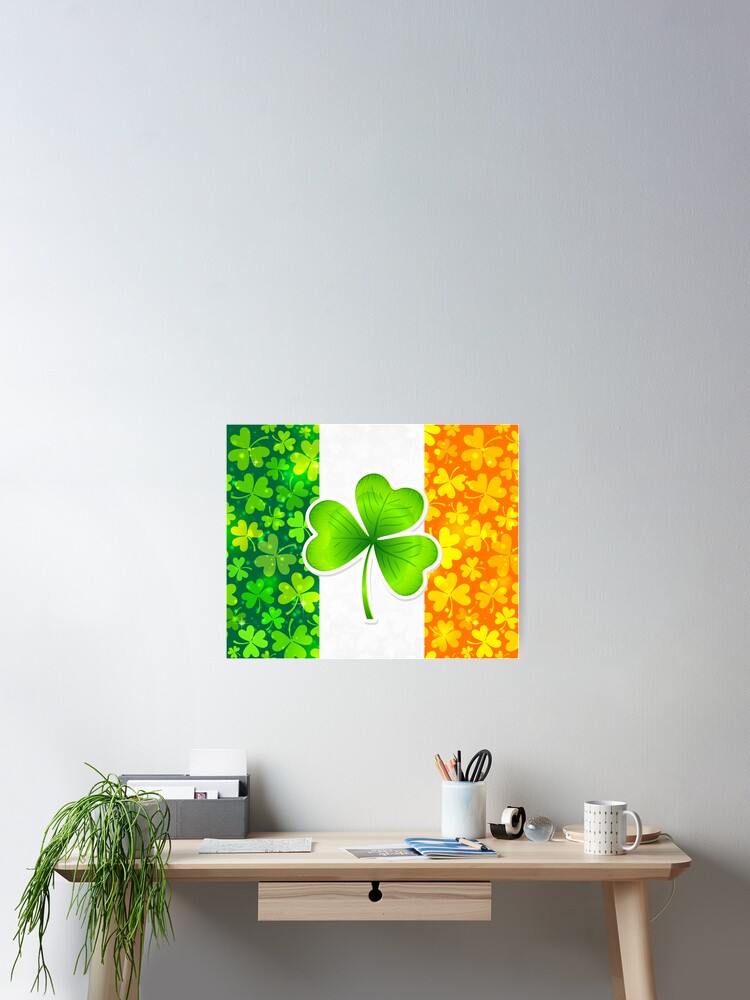The image depicts a room with a white wall, featuring a prominent picture of the Irish flag adorned with numerous three-leaf clovers. The flag, with its green, white, and orange vertical stripes, includes many small clovers in both the green and orange sections and a single large clover in the central white section. Below the flag is a small, tan-colored wooden desk with a single drawer. On the left front corner of the desk sits a green potted plant with long, stringy leaves. The desk surface is organized with various office supplies: on the left, there’s a paper bin; in the center, a white jar filled with scissors, pens, and pencils; a tape dispenser; and on the right, a white adjustable lamp, a white coffee mug, and some papers and booklets. The entire setup has a minimalist yet functional aesthetic, possibly indicating a workspace within a home environment.